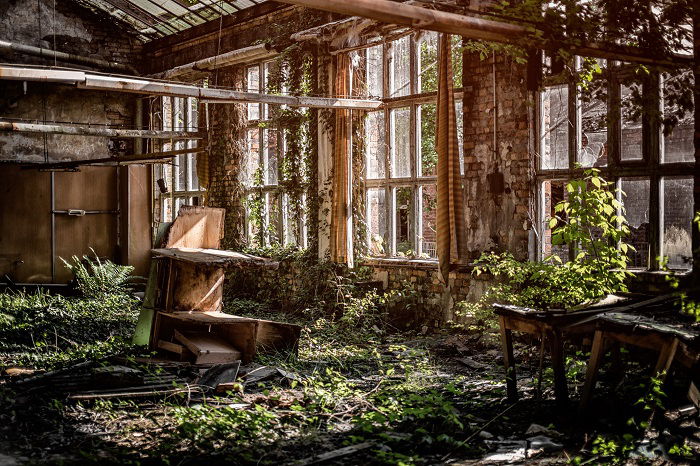The photograph showcases the interior of an abandoned building or house engulfed in decay and nature's reclamation. The room features very tall, brick walls, with four large windows stretching from about two feet above the floor to the ceiling, many of which are broken and draped with old, tattered curtains. The windows and damaged ceiling, punctuated with rusty, broken fluorescent light panels hanging precariously, hint that the space might once have been a classroom or possibly a greenhouse. The interior is almost completely overgrown with vines and various plants, blurring the lines between indoors and outdoors. Exposed conduits snake up the weathered walls, adding to the sense of ruin. Scattered throughout the room are shattered desks, broken wooden furniture, and remnants of what could have been grow benches, underscoring the room's dilapidated state. This abandoned, ruined sanctuary tells a haunting story of neglect and nature's persistent encroachment.